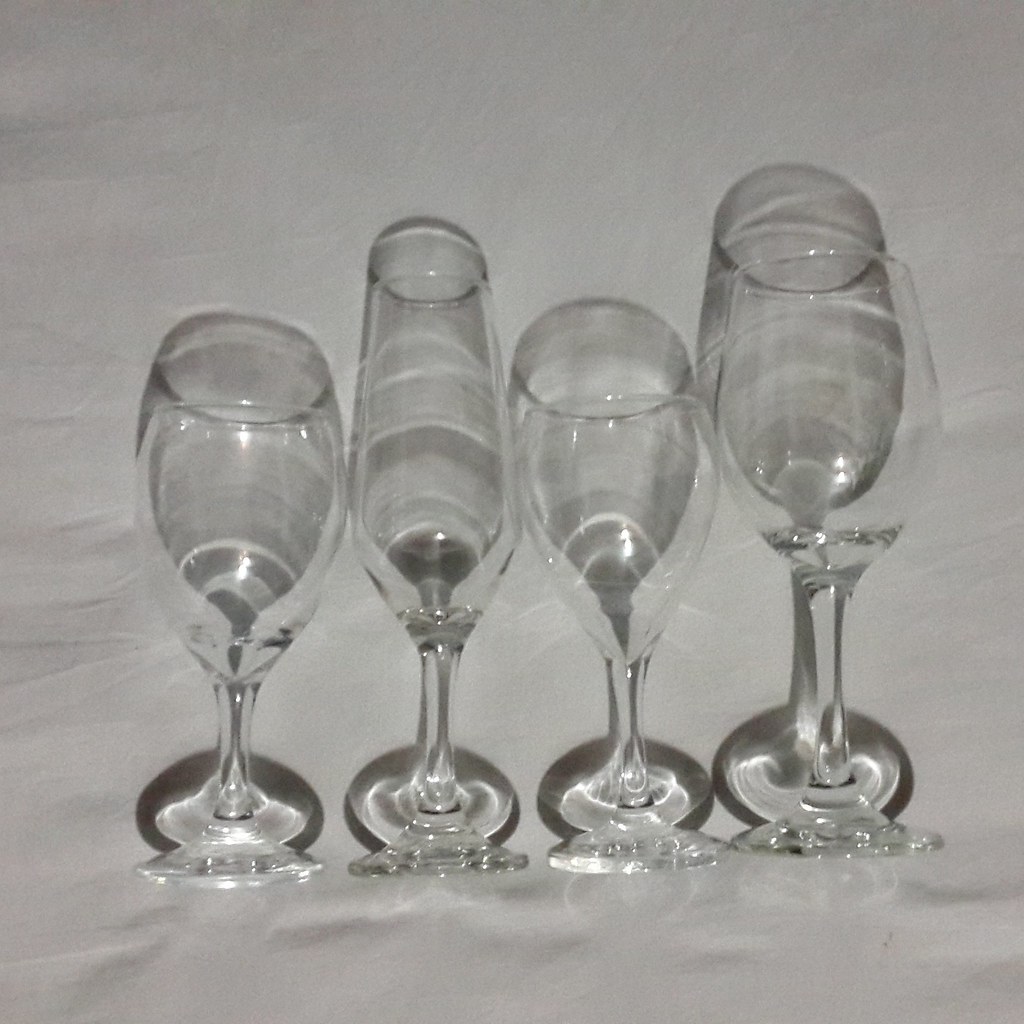This is a detailed photograph of four clear stemmed glasses arranged in a row from left to right on a white tablecloth. The order of the glasses alternates by height: a shorter wine glass, a taller fluted champagne glass, another shorter wine glass, and finally a taller wine glass. Each glass has a bulbous bowl and appears highly polished, reflecting light. The tablecloth beneath them reveals slight ripples and bumps. Additionally, elements behind the glasses, possibly a mirror, reflect their bases encircled by black shadows, creating a unique optical illusion where the reflections seem integrated with the glasses, almost distorting the view and necessitating a second look to comprehend the scene fully. The entire setting is bathed in light, which could be from a camera flash or direct illumination, further emphasizing the delicate contours of each glass.